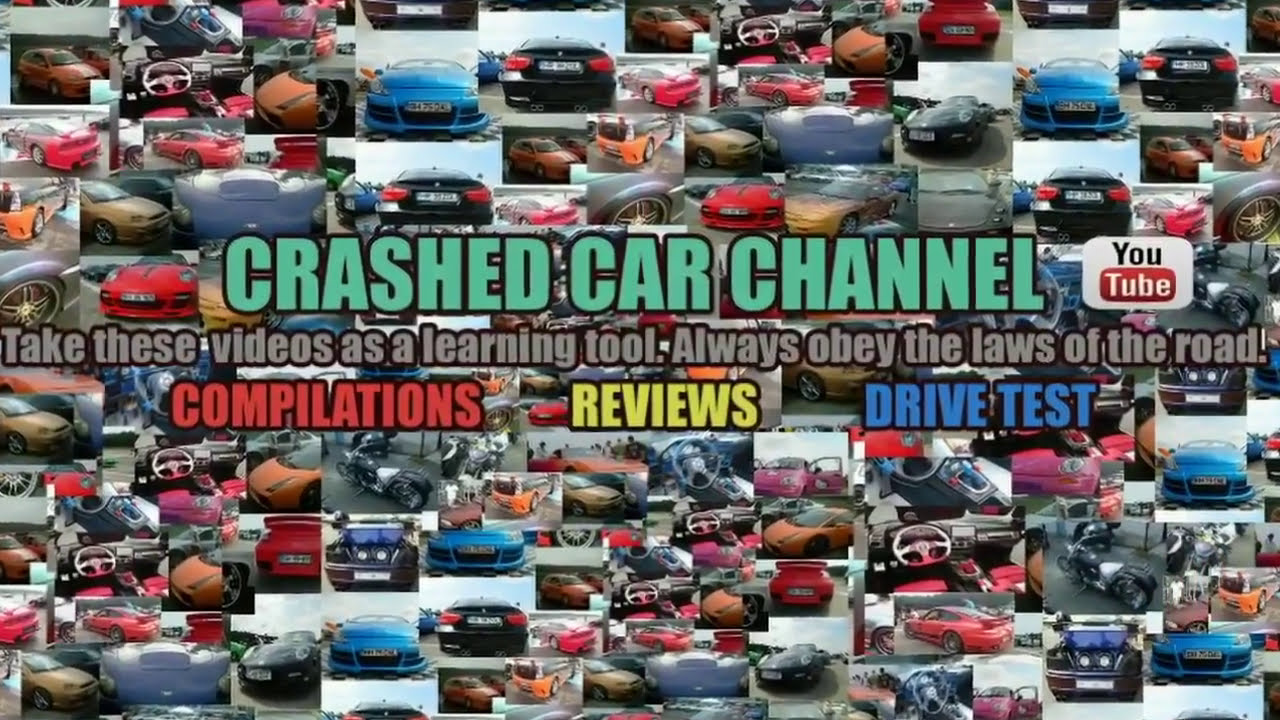The image is a vibrant and detailed banner for a YouTube channel named "Crashed Car Channel." The background is densely packed with a myriad of car pictures showcasing different angles and close-ups, including wheels, bumpers, and overall views. The cars vary from classic models like a '65 Mustang to modern supercars such as Ferraris, Lamborghinis, Porsches, BMWs, and Mercedes, all bearing European license plates. The center of the image prominently features large text in blue that reads "Crashed Car Channel," accompanied by the YouTube logo, which shows "You" in black and "Tube" in white encapsulated in a red rectangle. Beneath this, in gray text, it advises, "Take these videos as a learning tool. Always obey the laws of the road." Further down, it offers content details: "Compilations," "Reviews," and "Drive Test" in red, gray, and blue, respectively. The image is bright and colorful, dominated by hues of red, orange, yellow, blue, purple, green, pink, white, black, gray, and gold, and is indicative of the eclectic and informative nature one would expect from the YouTube channel it advertises.